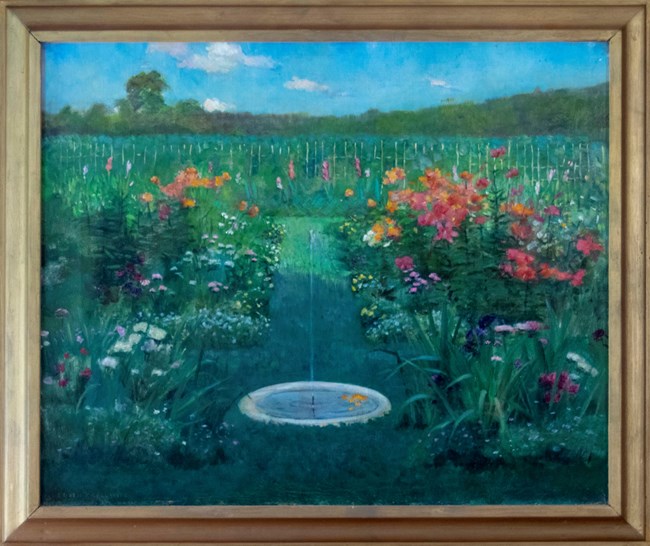This detailed painting, encased in a shabby chic wooden frame, depicts a serene garden scene. In the foreground, a small water fountain with a thin jet that fans out gracefully catches the eye, with a single fish, likely a goldfish or koi, swimming within. Surrounding the fountain, a profusion of vibrant flowers in hues of red, orange, pink, white, and purple, along with overgrown vegetation, spreads across the scene. A narrow grass pathway meanders through this lush garden, leading to a background fenced area ensconced in greenery and trees. Above, a clear blue sky is dotted with a few fluffy clouds, completing the tranquil atmosphere of this oil painting.